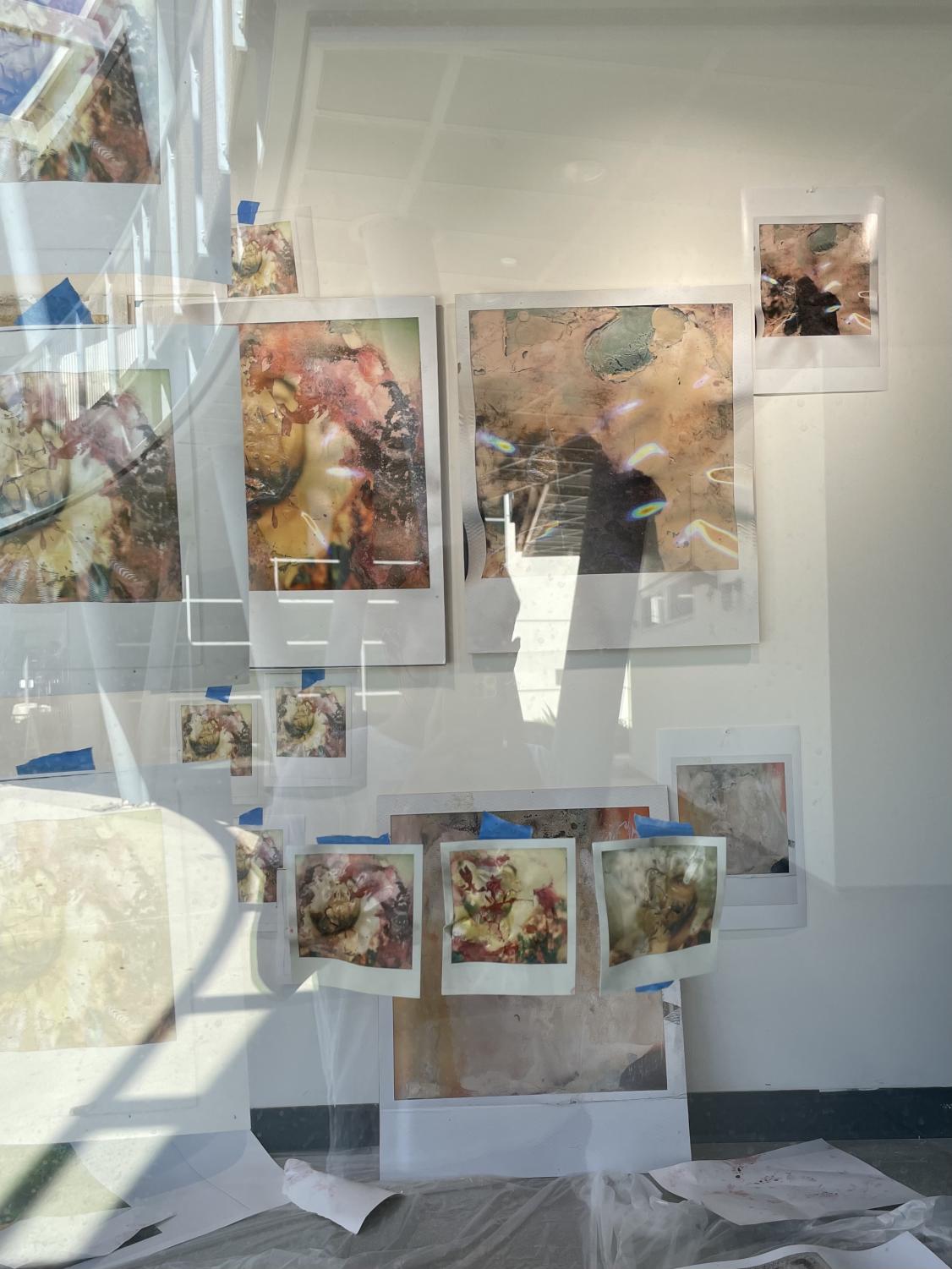This detailed photograph captures a scene viewed through a pane of glass at street level, likely into an art gallery or display window, characterized by its interesting play of reflections and direct views. The primary focus appears to be a collection of artwork, predominantly printed on white sheets of paper and mounted on a white wall with blue painter’s tape. These artworks include a mixture of mythical figures, aerial shots, and close-ups of flowers and plants, arranged with three larger central pieces surrounded by several smaller ones. Some artworks are still resting on the floor, yet to be hung. The glass provides a secondary layer of complexity by reflecting the scene behind the photographer, which includes a ceiling, possibly a staircase, a pillar, and even a second-story balcony from an external building. The predominant colors within the photograph are the white of the walls and paper, paired with subtle hints of pinks and light tans, making it challenging but intriguing to distinguish between the actual artworks and their reflections.